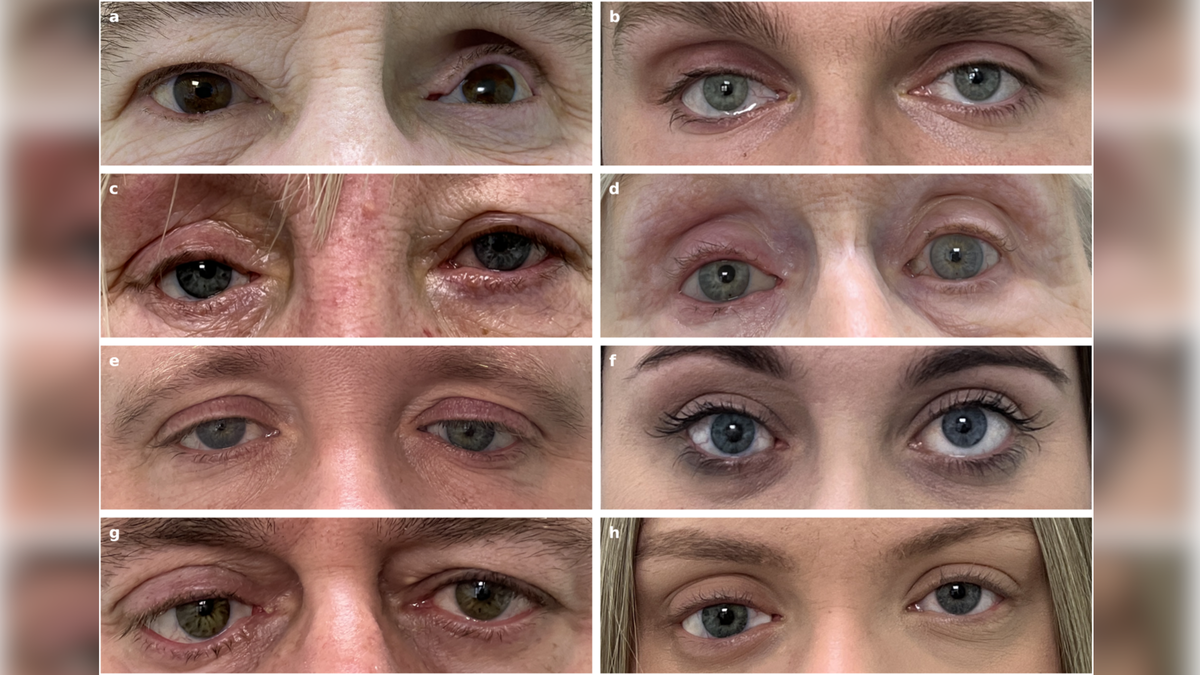The image presents an array of close-up photographs featuring the eyes of eight individuals, labeled from A through H. Each individual shares a beige, European-like skin tone. The focus is solely on the eyes, allowing for the observation of various eye and hair colors, as well as the differing shapes and features of the eyes. 

In image A, we see an older woman with brown eyes, where one eye appears smaller than the other. Image B features greenish-blue eyes belonging to someone whose eyes look slightly watery and differently shaped. Image C is of an older man with blue eyes, and image D shows an older woman with blue-green eyes. Image E depicts a man with blue, somewhat droopy eyes. Image F shows a woman with blue eyes, one slightly higher than the other. Image G belongs to someone with green eyes, likely a man. Lastly, H features a woman with blue eyes, with one eye appearing slightly smaller.

The series highlights the diversity in age, eye color, and asymmetry among the individuals, framing the subtle imperfections and unique characteristics of each set of eyes. The photos are cropped to display their eyebrows, eyes, and part of the bridge of their noses while including slight glimpses of their hair.